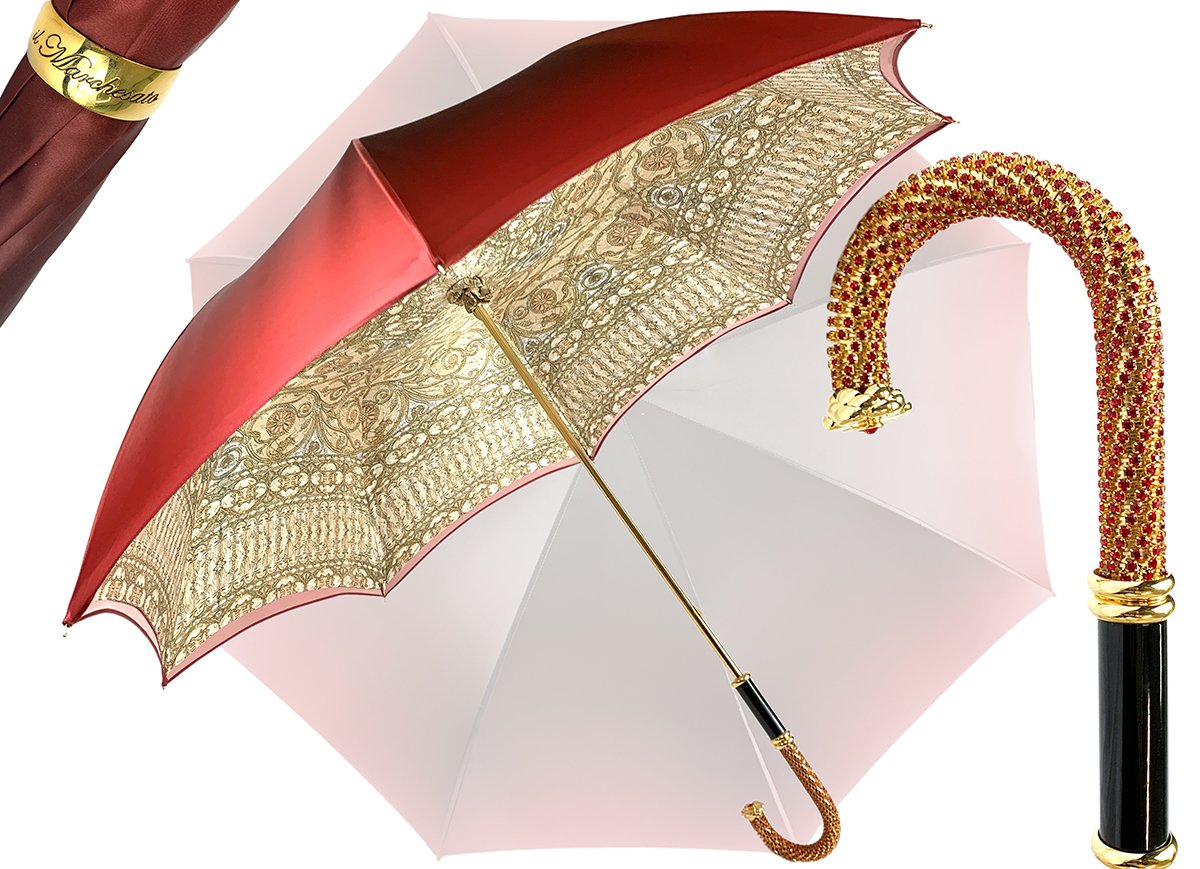The image features a highly detailed and elegant red umbrella with a luxurious gold underside. The umbrella has a maroon cloth cover in the top left corner, wrapped in a gold band. A significant aspect of the image is the close-up view of the umbrella handle, shaped like a candy cane, adorned with ruby red jewels and golden trim, enhancing its classy and sophisticated appearance. The main shaft of the umbrella appears to be gold, contributing to the overall opulent design. Inside the umbrella, intricate gold embroidery is visible, adding to its lavishness.

Additionally, the image shows a gold cane-like handle with a black cylindrical section featuring gold accents. This cane handle curves gracefully, complementing the umbrella's aesthetic. Engravings are present on a gold band of the cane, hinting at a potential brand or artist signature. A faded purple-toned umbrella can be seen in the background, adding depth to the scene. The combination of rich colors, textures, and luxurious materials creates an exquisite and visually striking image.